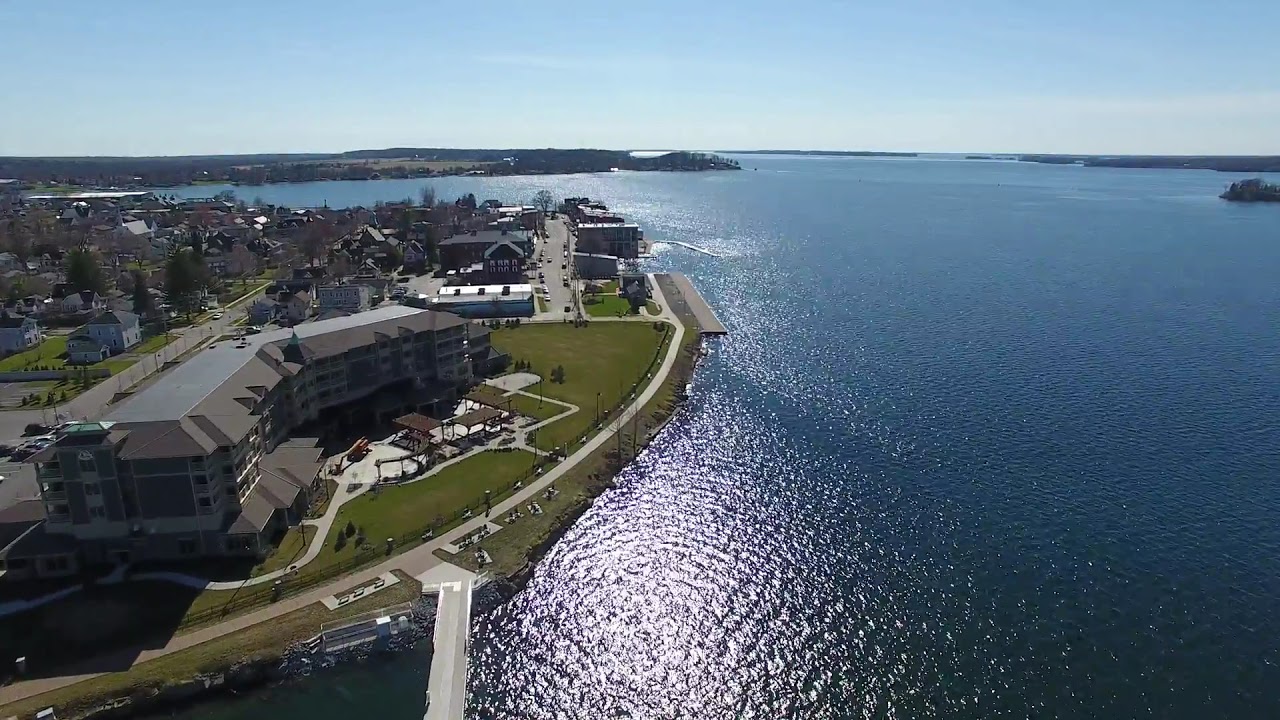This aerial view captures a stunning coastal cityscape and deep blue ocean, taken from an elevated vantage point. On the left side of the image, the bustling city stretches out with numerous buildings, roads, and a notable large structure that appears to be a hotel or apartment complex. This building is surrounded by a well-manicured grassy area and features various cement sidewalks and covered picnic spots, enhancing its inviting ambiance. Further up the coast, a collection of smaller buildings and shops lines the waterfront, adding to the vibrant urban scene.

To the right, the serene ocean extends into a calm bay, its dark blue waters reflecting the sunlight and presenting a tranquil, wave-free surface. A small island and several land features punctuate the coastal waters, adding geographic diversity to the scene. Above, the clear sky is a light blue with a few wispy clouds, indicating a beautiful and sunny day. This image captures a harmonious blend of urban development and natural beauty, showcasing the dynamic interactions between land and sea.